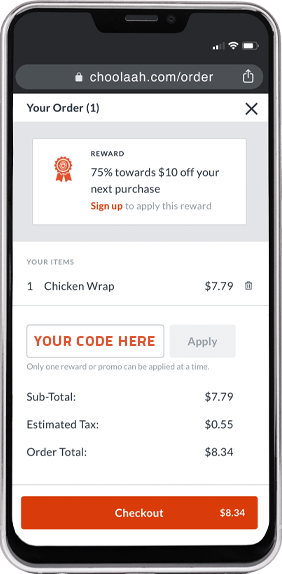The image appears to be a screenshot of a mobile phone screen mock-up, characterized by a polished, silver rounded edge and an iPhone-style notch at the top center. Despite its realistic elements, it doesn't look entirely photorealistic. The screen displays typical phone status icons in white on the right side of a black top bar: two bars of mobile signal, three bars of Wi-Fi signal, and a full battery charge icon.

Below this, there's a grey search box featuring a padlock icon and the URL "chula.com/order." The main content area has a greyish or white background. On the left, the text "Your order" appears in black with "(1)" beside it, and an "X" symbol for closing the order summary on the right.

Further down, a grey bar holds a rectangular notification that reads: "Reward 75% towards $10 off your next purchase," highlighted by a red reward ribbon on the left. The text "Sign up to apply this reward" is also visible. 

Continuing below this section, details of an order are provided. The item listed is "Chicken wrap," priced at $7.79. Below this, there's a red prompt saying "Your code here" next to a box for entering a promotional code, with an "Apply" button in grey to the right. A note indicates that only one reward or promo code can be applied per order.

The cost breakdown includes a subtotal of $7.79, an estimated tax of $0.55, leading to a total order amount of $8.34. At the bottom, there's a prominent red "Checkout" button spanning the width of the screen, featuring the total amount "$8.34" on the right side in white text.